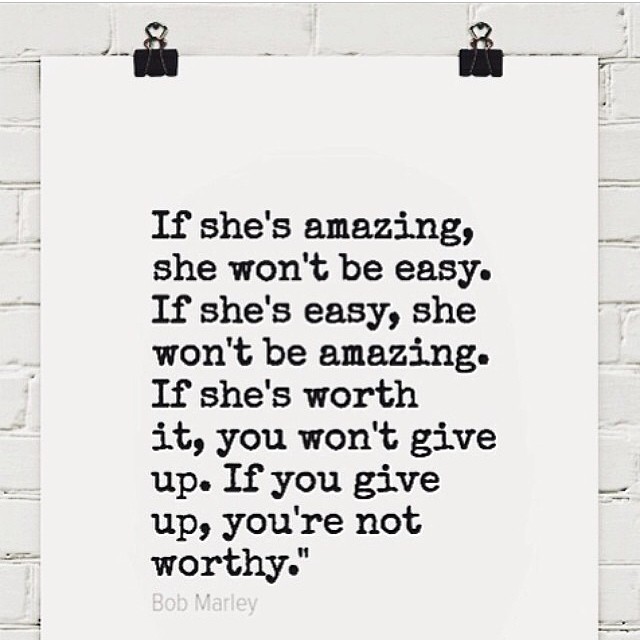In this image, a white painted brick wall serves as the background, against which a piece of paper is prominently displayed. The paper is clipped to the wall with two black metal paperclips positioned at the top left and top right corners. Centered on the paper is a motivational message printed in black text that reads, "If she's amazing, she won't be easy. If she's easy, she won't be amazing. If she's worth it, you won't give up. If you give up, you're not worthy." Below this, in a much lighter gray text, is the attribution "Bob Marley." The short quote spans nine lines, evenly spaced and neatly aligned. There are no other objects or elements in the image, giving it a clear and focused aesthetic. The overall style suggests that this is a social media meme, designed to share an inspirational message about relationships.